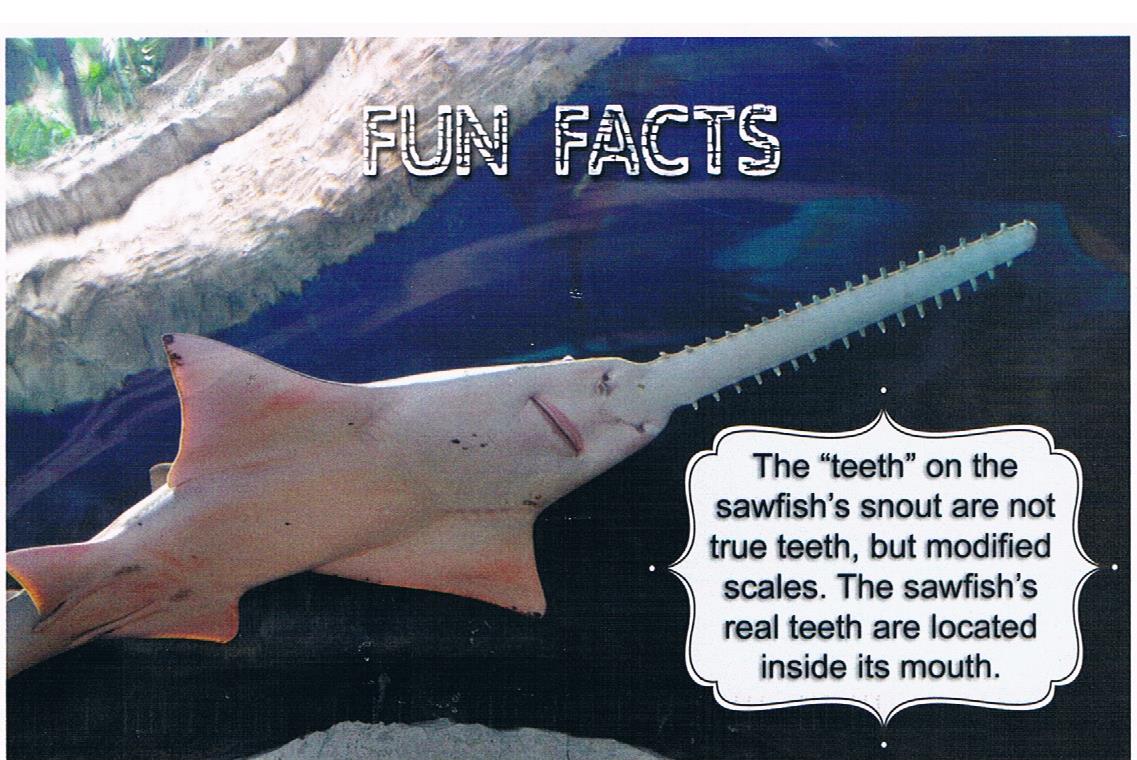The image features a distinctive sawfish, depicted from a unique bottom view, with its pink body and white saw-like snout. Above the sawfish, rocks can be seen, giving the impression that the creature is swimming along the ocean floor. The background includes a blue area interspersed with gray sections representing sandbanks, adding to the underwater ambiance. 

At the top of the image, the phrase "Fun Facts" is prominently displayed in white-bordered letters. In the lower right corner, a white balloon or bubble contains informative black text, stating: "The teeth on the sawfish's snout are not true teeth, but modified scales. The sawfish's real teeth are located inside its mouth." This educational note serves as an intriguing insight into the biological features of the sawfish.